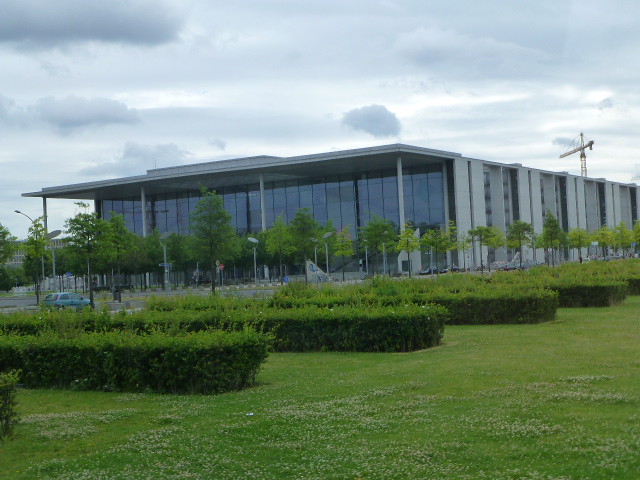This photograph captures a large, modern rectangular building, prominently featuring a front facade made entirely of glass panels while the sides are constructed from light-colored stone. The structure is accented with a roof supported by four posts matching the stone sides. Specific attention to landscaping is evident: a well-manicured, expansive lawn occupies the foreground, dotted with meticulously spaced rectangular bushes and evenly planted matching trees that extend into the distance. Adding to the structured appearance, a single teal-colored sedan is parked mid-left, providing a sense of scale. To the right of the building, a construction crane is visible, hinting at ongoing development. The sky overhead is filled with thick, gray clouds suggesting imminent rain, and the daytime lighting casts a diffused glow across the scene.